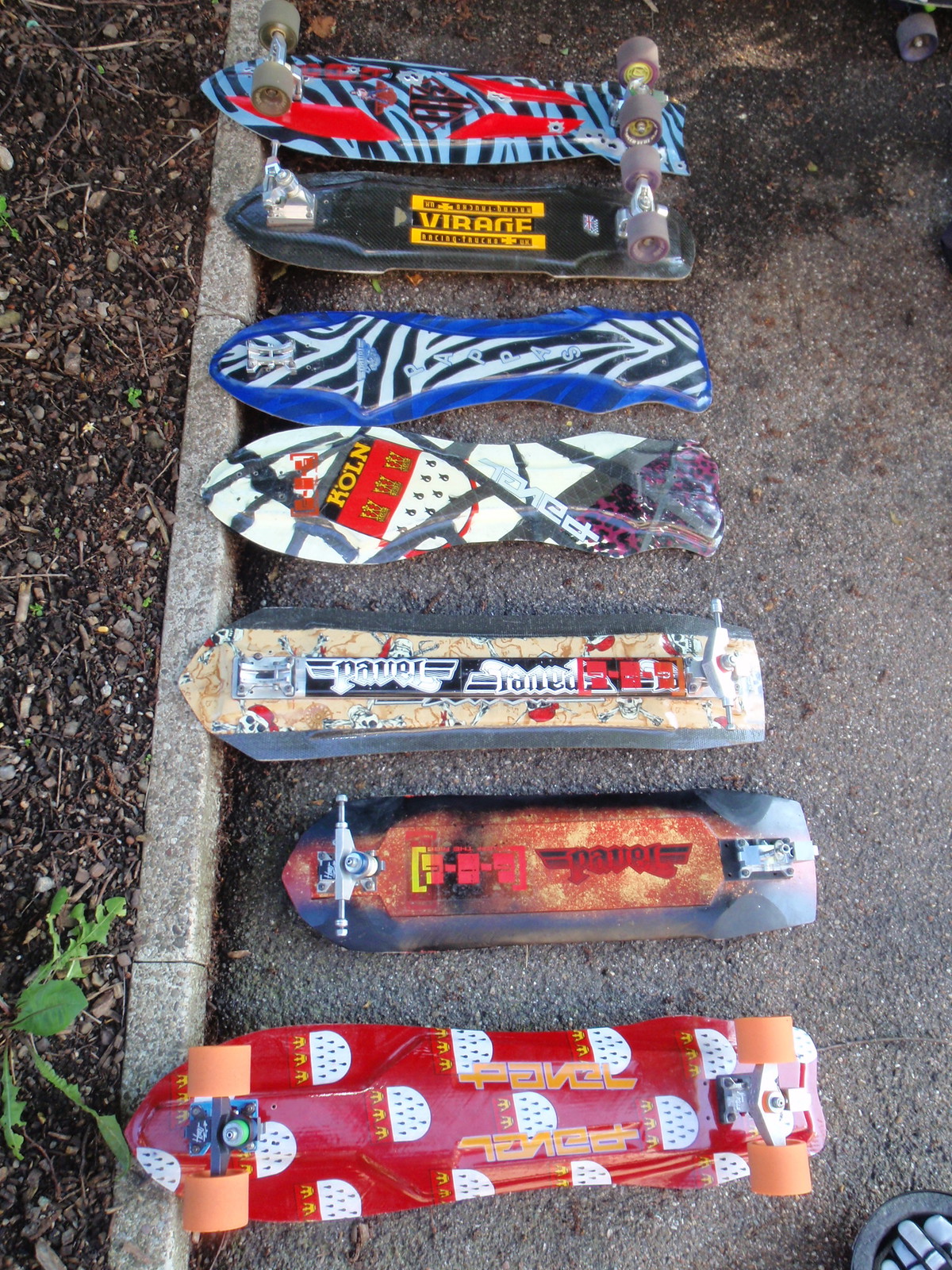This outdoor photograph captures an array of seven skateboards arranged on a cement pavement, bordered by a small curb on the left, adjacent to a sparsely vegetated area with soil, scattered stones, and green sprouts. The boards display a vivid variety of designs and conditions.

The first skateboard, positioned with its front end on the curb, features a prominent red and orange bottom with peach-colored wheels and the barely legible text "PAVEL" in unusual lettering. There are abstract black, white, and yellow shapes as part of the design.

The second skateboard, slightly smaller, is missing its rear truck and has no wheels. Its design includes a red, flame-like motif encased in black, with indistinct red text that might read "PAVEL" or "PAVER."

The third skateboard showcases a pirate theme with skulls and red bandanas, over a tan background bordered by black lines. The text, likely "PAVER" or "PAVEL," appears twice, though one truck is missing while the other lacks wheels.

The fourth board is completely stripped of trucks and wheels, boasting a chaotic pattern of colorful lines and small designs. Noteworthy is the text "KOLN" and distinctive sections of red and black squares accentuated by yellow writing.

The fifth skateboard is adorned with a blue-trimmed, zebra stripe design and also lacks trucks and wheels. A difficult-to-read inscription might say "PAPRAS".

The sixth skateboard, predominantly black, has a unique yellow and black bar pattern with alternating colored text. Words inscribed in yellow on the black bar spell out "VIRAGE." It has both trucks intact, though only the rear truck has wheels.

The seventh and final skateboard features blue and black zebra stripes with red shapes, and a conspicuous red and black logo at its center. It retains all its trucks and wheels.

The overall setting appears to be a park or a parking area, with the skateboards laying on a faded, dirty concrete surface that may have marking shadows or oil stains. The scene exudes a casual, almost forgotten air, as if the skateboards were spontaneously left behind amidst play.